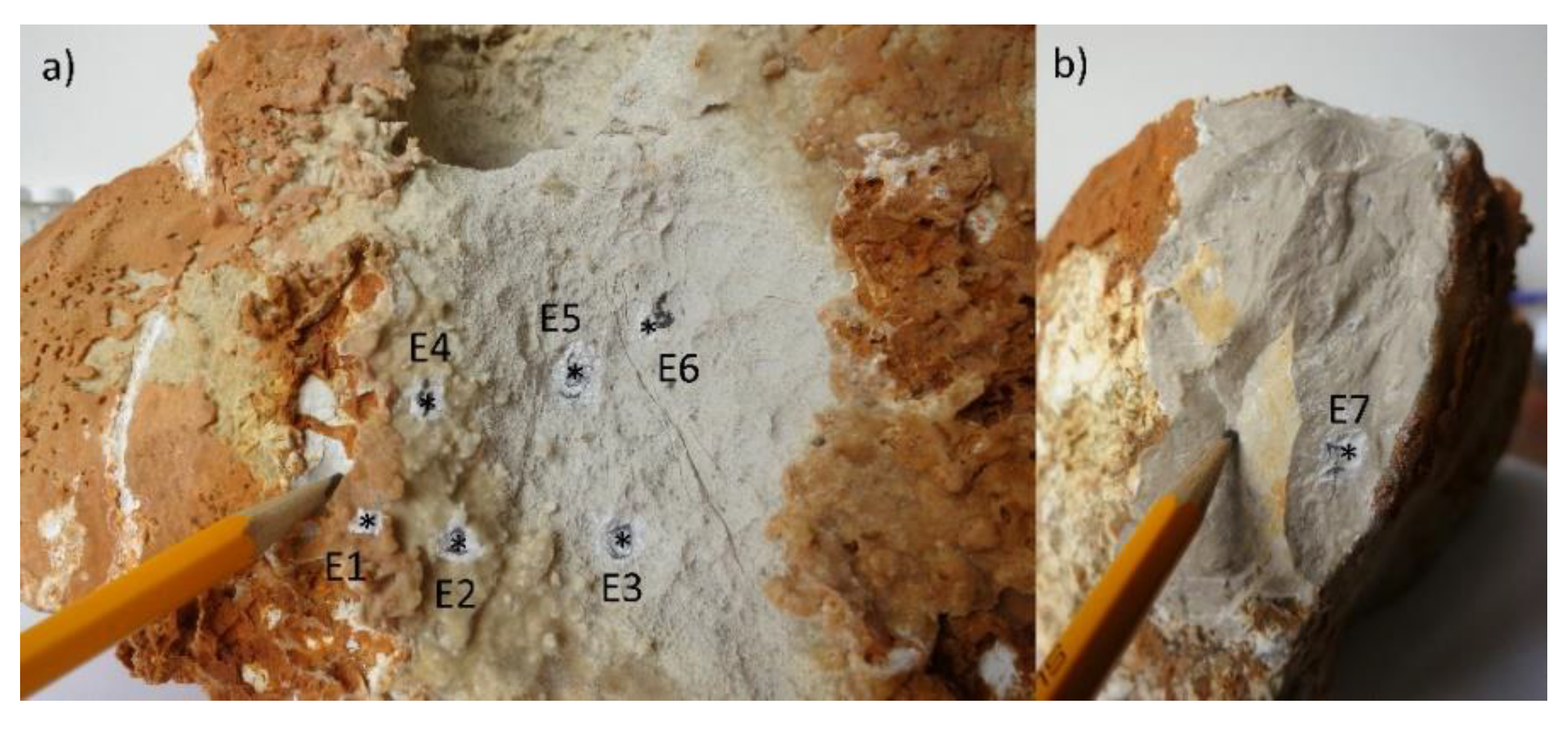This side-by-side photograph showcases close-up images of a highly porous rock formation or mineral specimen, with the image on the left labeled as "A" and the one on the right labeled as "B." In photograph A, six small, star-shaped inclusions are highlighted and labeled as E1 through E6. Accompanying these labels is a yellow pencil, pointing towards these inclusions to provide size and scale. The rock appears reddish with areas of white erosion and numerous porous sections, resembling a sponge cake in texture. In photograph B, the same type of mineral or rock is displayed, featuring a single labeled inclusion, E7. A yellow pencil is similarly positioned in this image to indicate size, pointing at a pinhole or chip in the mineral. Overall, both photos detail the intricate and eroded surface of the rock formation, marked with specific points of interest.